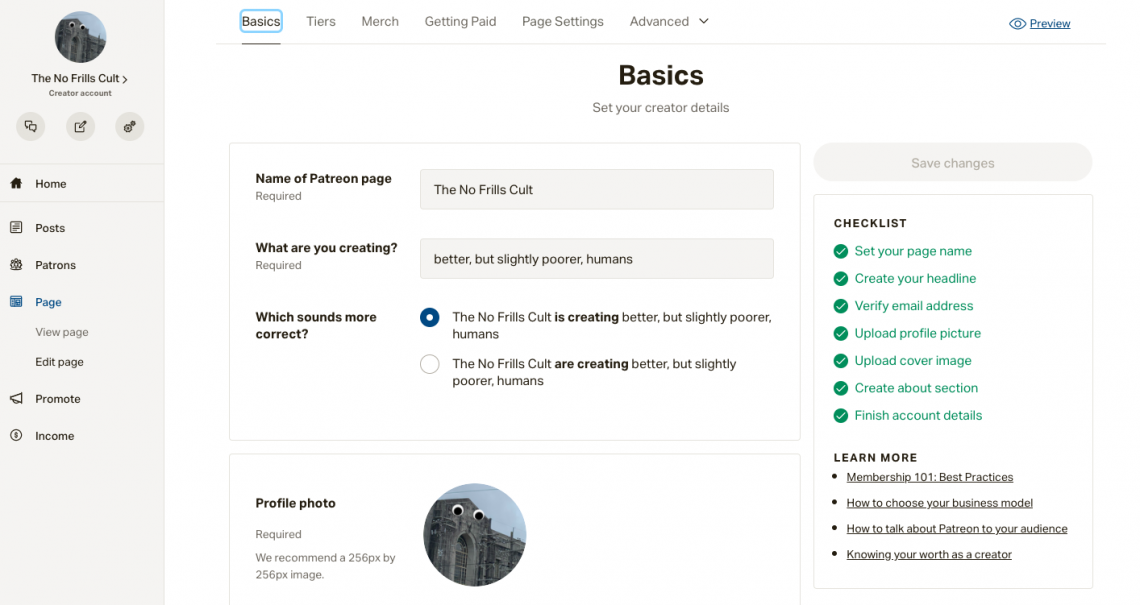### Detailed Caption:

The image depicts a settings page on Patreon for the "No Frills Cult," a creator account. At the top of the page, there are tabs labeled "Basics," "Tiers," "Merch," "Getting Paid," "Page Settings," and "Advanced," suggesting this is an administrative area for configuring a Patreon page. The page title, "No Frills Cult," is prominently displayed, and the profile photo features an image of an old building adorned with googly eyes, adding a quirky touch.

On the left side of the screen, a navigation pane lists options such as "Posts," "Patrons," "Page," "Edit Page," "Promote," and "Income." To the right, a comprehensive checklist indicates that the creator has completed various setup tasks, including setting the page name, creating a headline, verifying the email address, uploading a profile picture, uploading a cover image, creating an about section, and finishing account details.

Below the checklist, additional resources are provided, such as "Learn More," "Membership 101," "How to Choose Your Business Model," and "Knowing Your Worth as a Creator." The background of the page is white, and most of the text is in black, maintaining a clean and minimalistic design. Overall, the image captures the detailed settings interface where creators manage their Patreon accounts.